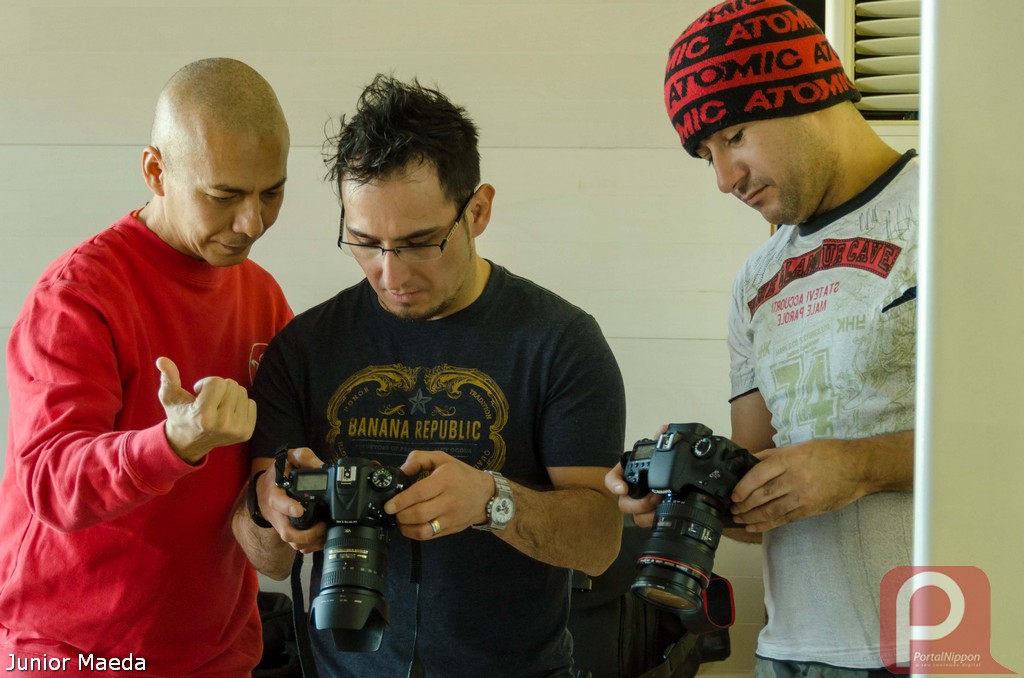In this detailed photograph, three men are seen standing inside a room, each absorbed in examining their own cameras. The man on the left is bald and is dressed in a red, long-sleeve shirt. He is attentively gazing at the camera held by the man in the middle. The middle man, who has slightly messy short black hair, wears glasses and has a bit of facial hair on his chin. He's sporting a black, short-sleeve t-shirt emblazoned with "Banana Republic" in gold lettering, along with a silver wristwatch and a wedding band on his left ring finger. He is closely inspecting a large black camera with a substantial lens. The man on the right is also occupied with his camera; he is wearing a white short-sleeve t-shirt featuring some design, and a distinctive red and black beanie with the word "Atomic" repeated on it. Behind the trio, the wall is painted white and features a window on the top right side. Notably, the bottom left corner of the image contains the words "Junior Maeda," and the bottom right corner showcases a logo with the word "alphabet P."